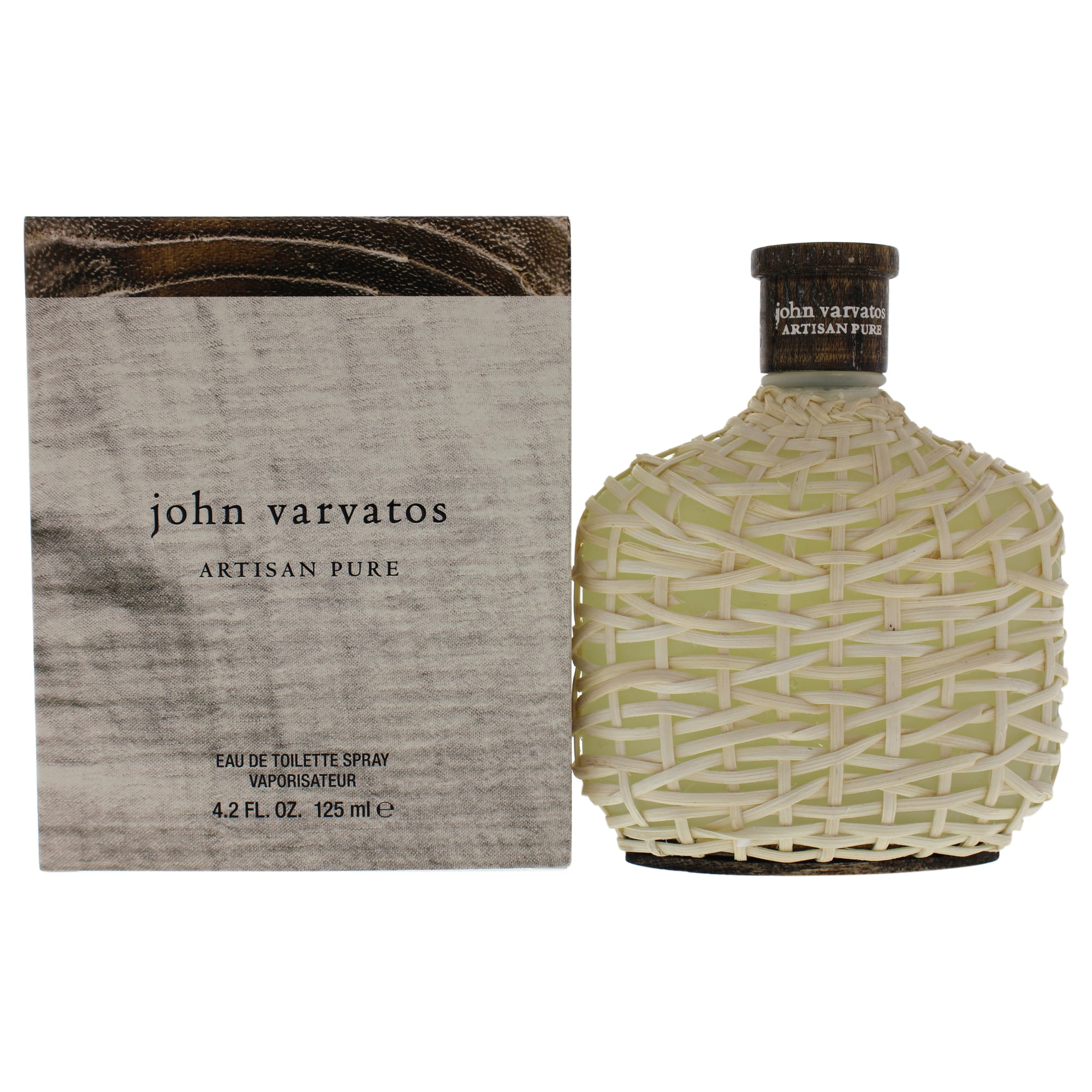The detailed close-up image showcases a John Varvatos Artisan Pure eau de toilette spray set. On the right, the distinctive glass bottle is adorned with an ivory cream-colored vine or twine wrapping, giving it a textured, natural appearance. The bottle features a dark brown, wooden-like cap and displays the branding "John Varvatos Artisan Pure." It also appears to be around four inches tall, in line with the packaging dimensions. To the left of the bottle is the coordinating box, a sturdy-looking package that reinforces the elegant, artisanal theme. It prominently states the product name and key details in both English and French, noting the contents as 4.2 fluid ounces (125 milliliters). The entire composition is set against a clean, white gradient background, accentuating the refined, earthy aesthetic of the items.